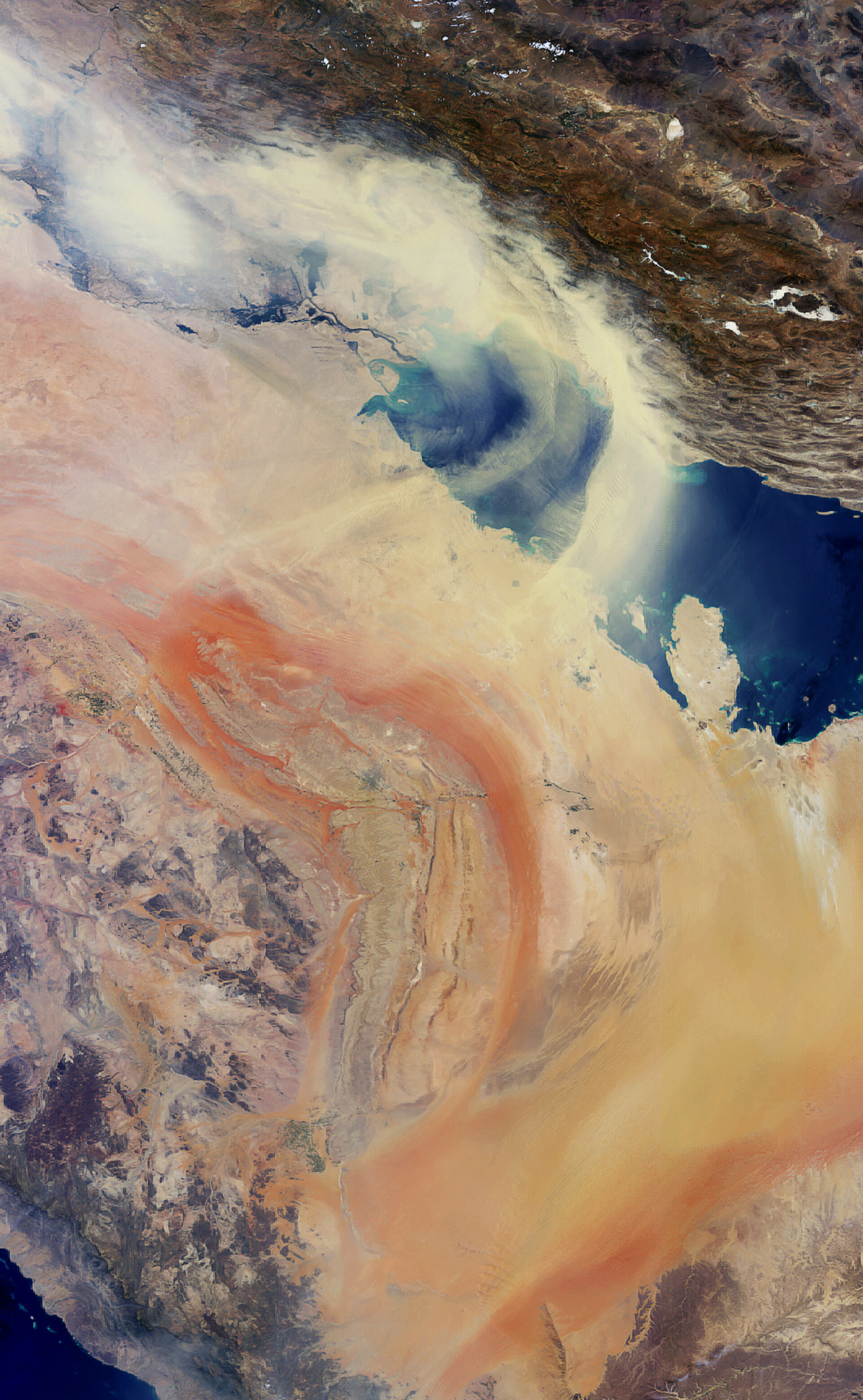The image presents an aerial perspective, capturing what appears to be an extraordinary view from an immense height, resembling airplane altitude, looking down on an intricate landscape. Starting approximately 20% down from the top of the image, a diagonal division marks the transition between two distinct sections. The area beneath this line on the left contains a light brown and orange-hued rocky terrain, likely indicative of a mountainous or canyon region, with swirling colors and a composition suggesting intricate geological formations.

A river-like feature separates this from the upper right section, which is characterized by a mix of green and light brown rocky textures. Further enhancing the surreal aspect, a pool of water or a similar reflective surface can be seen nestled between rock formations, with a wisp of clouds adding a dreamlike quality to the scene.

The upper portion of the image is dominated by very dark brown, almost spacey, wavy tones. Interspersed throughout, white and fluffy clouds flow through the entire composition, lending an ethereal, almost otherworldly, atmosphere. The bottom section showcases a blend of salmon, light tan, and white colors, gracefully intertwined.

Overall, the combination of these vibrant colors and diverse textures could suggest a highly detailed photograph from space or an artistic rendition of Earth's surface, where atmospheric elements such as clouds and intricate geological features merge into a captivating, colorful tapestry.